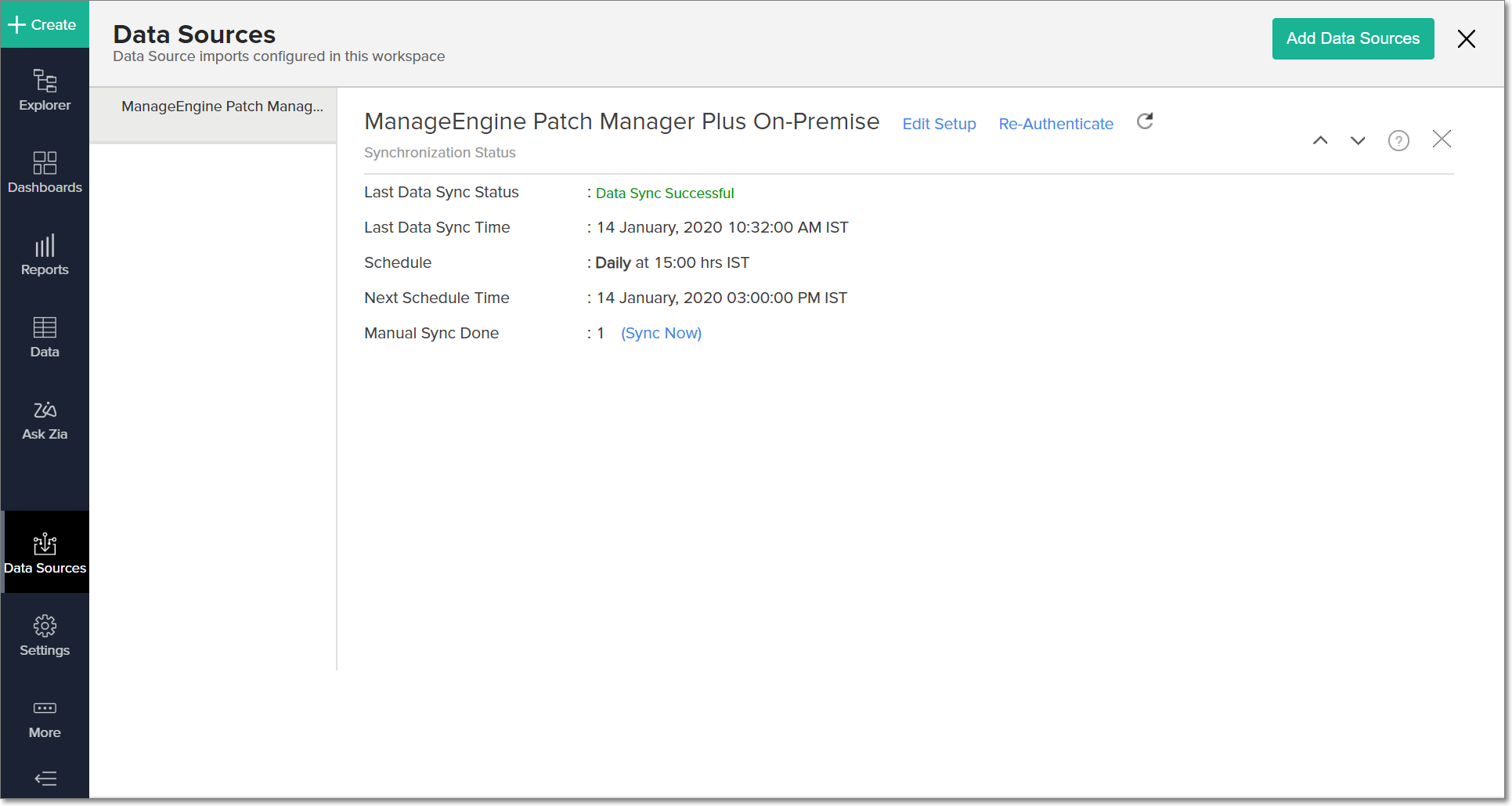This is a detailed caption based on the voice description provided:

---

This screenshot captures a browser window centered on the management of data sources. At the top, a prominently displayed title "Data Sources" is rendered in larger black text. Directly below, smaller text states, "Data Sources Import Configured in this workspace."

The far left side of the window features a black vertical navigation panel. This panel begins with a "Create" button at the top, followed by approximately ten icons: "Explorer," "Dashboard," "Reports" (depicted as bar graphs), "Data" (represented with a chart icon), "Ask Zia," "Data Sources" (illustrated as a box with an arrow pointing downwards), "Settings" (gear icon), "More," and a final icon consisting of three horizontal lines stacked vertically.

To the right of the navigation panel, the workspace is divided into multiple panes. The first pane bears the title "ManageEngine" (spelled as one word) followed by "Patch Manage." 

The subsequent, largest pane features a white background with the header, "ManageEngine Patch Manager Plus On-Premise." This section includes options for "Edit Setup," "Reauthenticate," and a refresh icon. Below these options is a list of data points:
- "Last Data Sync Status" noting "Data Sync Successful"
- "Last Data Sync Time" recorded as January 14, 2020, at 10:32 AM
- "Schedule," which is set to daily at 15:00 hours (3:00 PM)
- "Next Schedule Time," indicated as January 14, 2020, at 3:00 PM
- "Manual Sync," offering a "One Time Sync Now" action

This detailed configuration overview facilitates effective data management within the workspace.